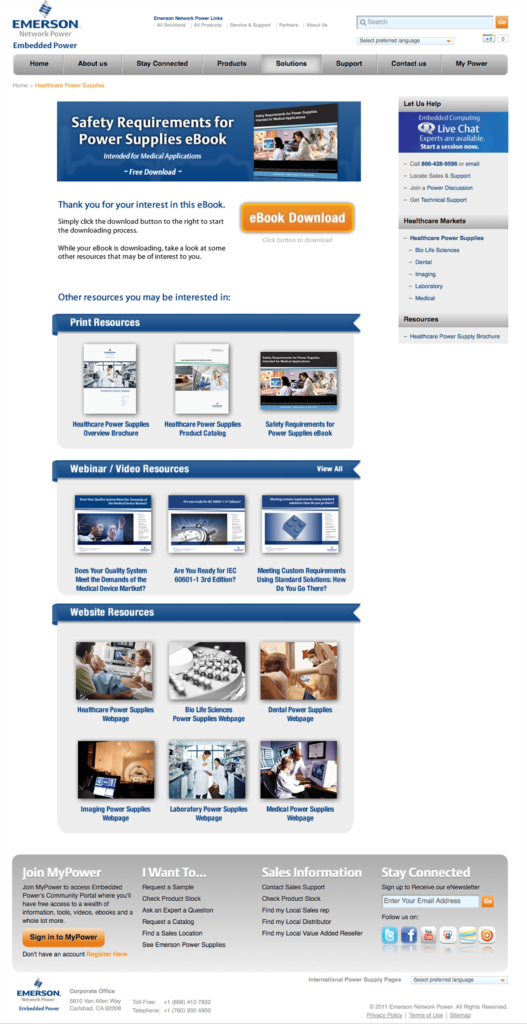This detailed webpage belongs to Emerson Network Power, a company focused on providing network power solutions. The website is designed for desktop viewing, with a prominent main menu featuring tabs such as Home, About Us, Stay Connected, Products, Solutions, Support, Contact Us, and MyPower, which is intended for user account management. The page currently displayed falls under the "Solutions" section, offering a comprehensive range of resources. These resources include an e-book download titled "Safety Requirements for Power Supplies," alongside various graphical elements, printed materials, webinar videos, and other types of content like PowerPoint presentations and infographics. While the specific details about Emerson's product offerings are unclear due to small and blurry text, the page is visually rich, aiming to provide extensive information and support materials.